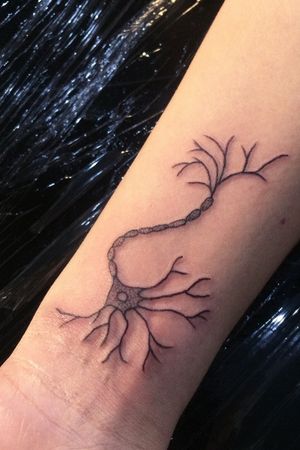The image showcases a freshly done tattoo on a person's wrist, which extends from just below the wrist wrinkles to about three-quarters up the forearm. The tattoo features a detailed, possibly scientific diagram with various elements. At the end near the elbow, there is a series of branching thin lines. These lines connect to a series of small, interconnected, pill-shaped ovals forming a chain that travels up towards the wrist. Higher up, closer to the wrist, there is a circular darkened area with a distinctive white circle in its center, from which more branching thin lines emanate. Scattered within the tattoo design are numerous dots. Notably, the person has a small freckle near the tattoo. The background is dark and glossy, resembling wet or gelled hair, adding a stark contrast to the well-lit Caucasian skin. The texture of the backdrop also resembles plastic fringes, contributing to an overall complex and intricate visual setting.